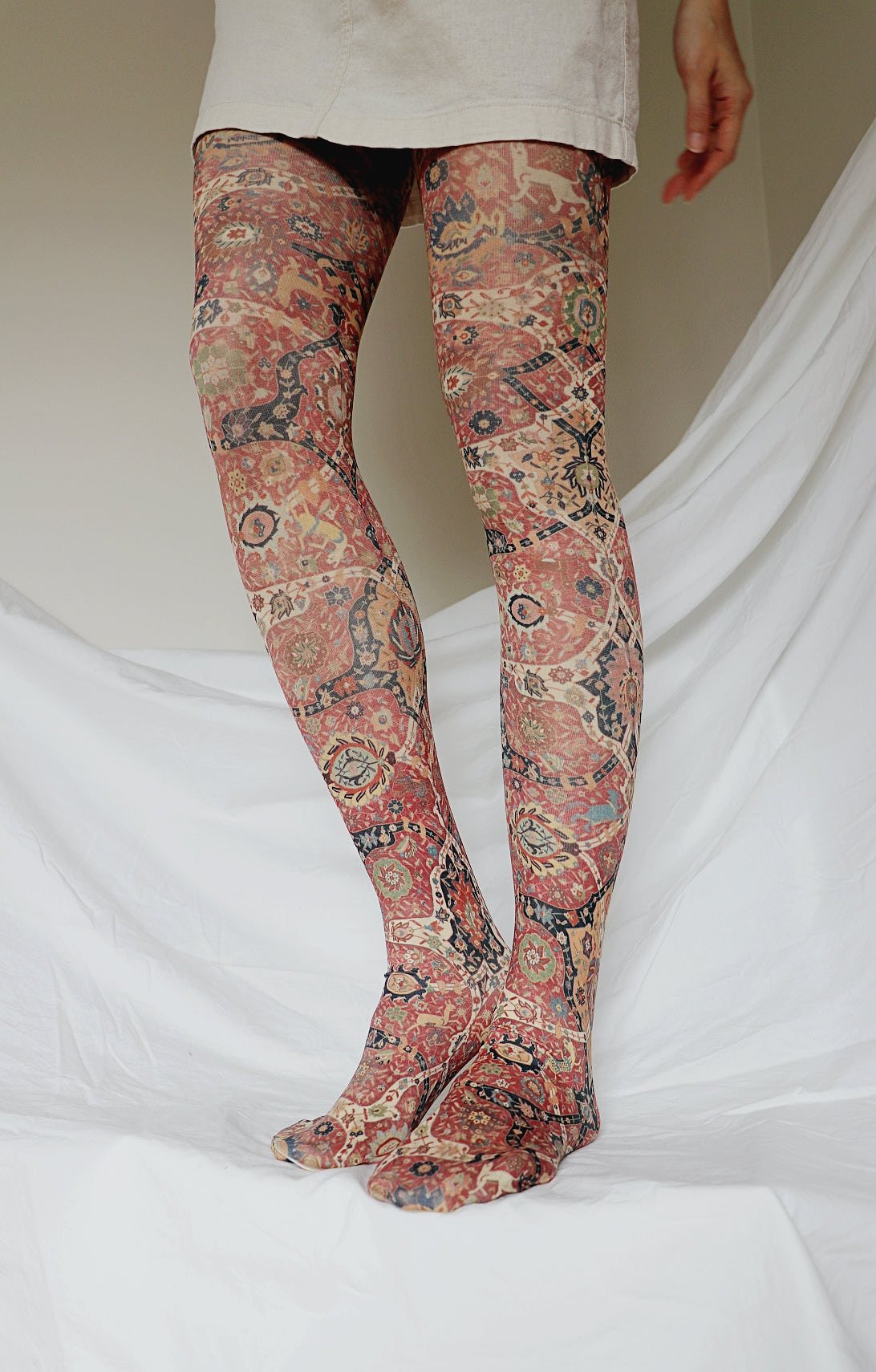The image depicts a woman standing on a white draped cloth against a cream white wall. She is wearing a short white skirt that falls to just above her knees, and her left hand is visible by her side, displaying a fair-skinned, feminine hand. The focus is on her legs, which are adorned in ornate nylon stockings. The stockings feature an intricate and elaborate design reminiscent of Persian rugs, with a predominantly red color punctuated by black lines, floral motifs, and abstract paisley patterns. Additional hues of blue, orange, yellow, and tan weave through the detailed patterns, enriching the overall vibrant effect. The white cloth she stands on arches downward past her knees, creating a soft, enveloping backdrop that complements the cream-colored wall.